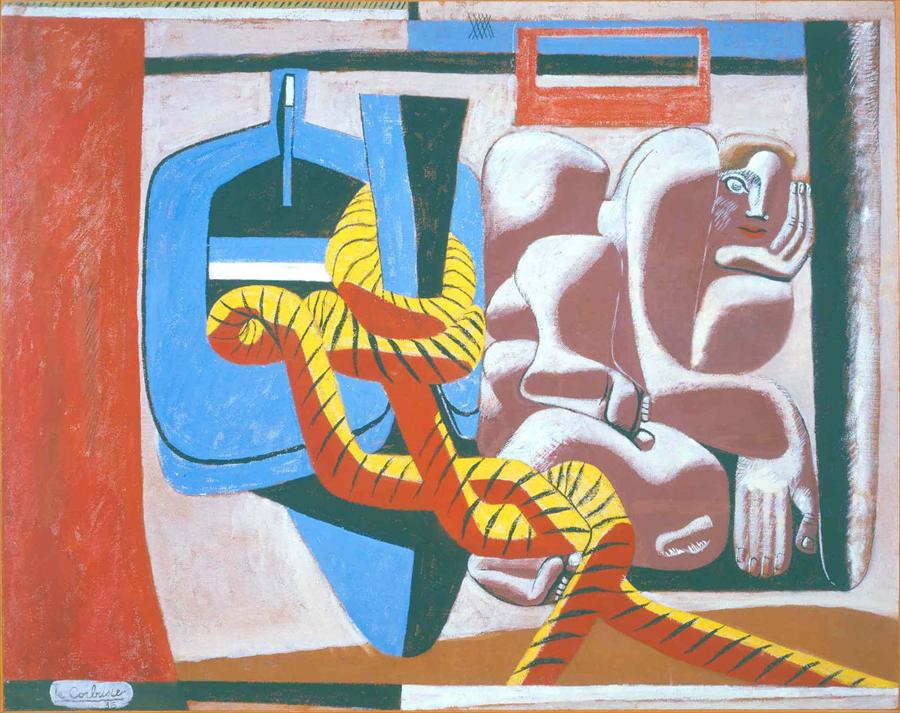This abstract painting, possibly created using chalk pastels or oil, showcases modern abstract art with cubist influences. Dominated by primary colors—red, yellow, and blue—it features a red brick-like panel on the left side, transitioning into various segmented shapes. A roundish blue cube-like form sits in the upper right-hand corner, entwined by a long, yellow snake-like or rope-like figure with black stripes. The centerpiece is a highly abstracted and fragmented human form, depicted with cubist techniques. This figure displays a jumbled collection of body parts—such as a shoulder, foot, hand, and facial elements like one eye, a nose, lips, and hair—layered atop one another. The color palette includes black, white, various shades of brown, off-white, and gold. In the bottom left-hand corner is a tiny, barely legible artist's signature, suggesting the painting might date back to 1935.